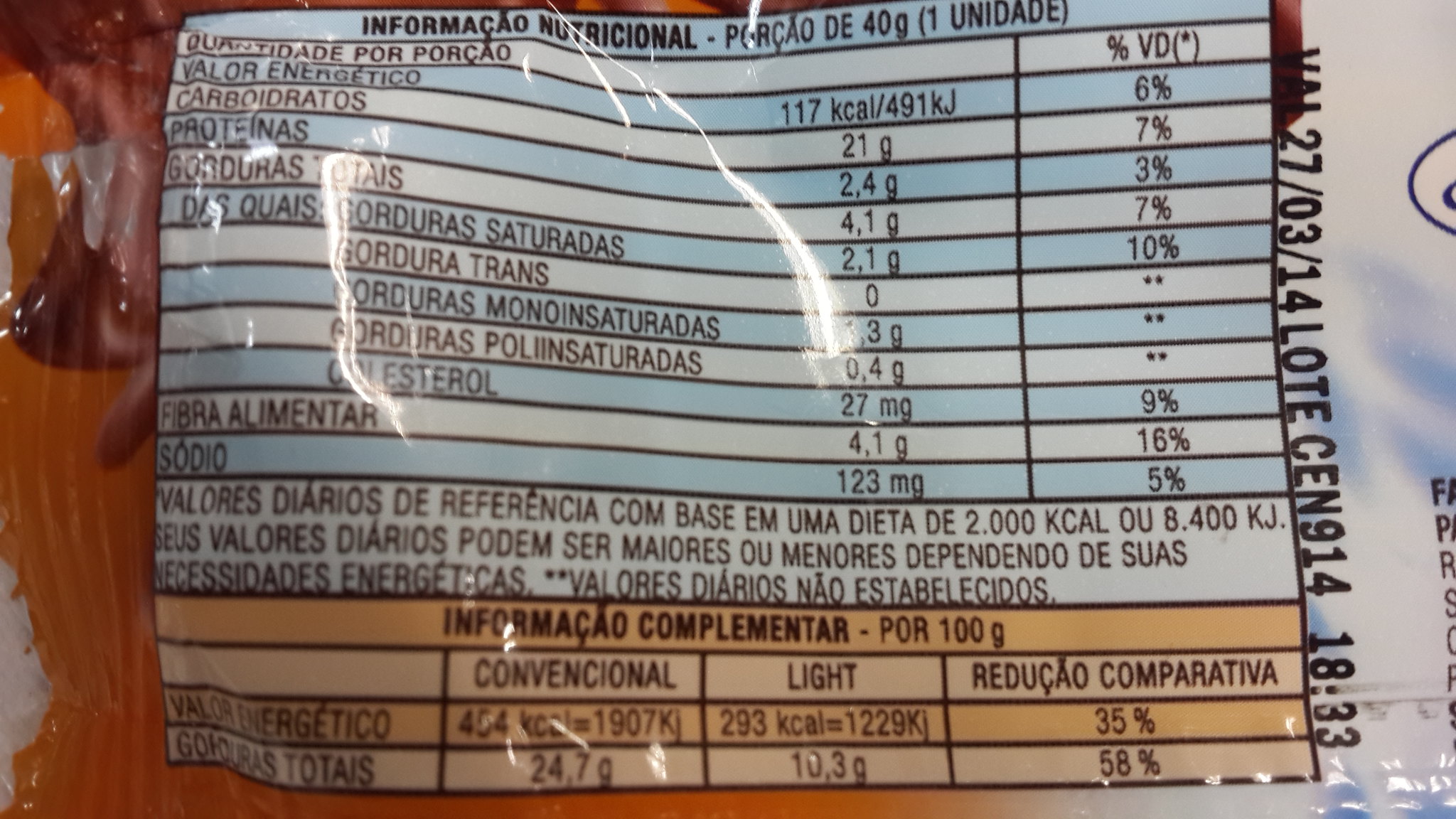The image depicts the back of a plastic-wrapped food package, likely written in Spanish. The label's top section is dedicated to nutritional information, formatted in alternating blue and light blue lines, listing components such as carbohydrates, proteins, fiber, and sodium. This section parallels typical U.S. labels, indicating values based on dietary needs. Below this, there's a complementary information chart in shades of orange, possibly detailing conventional, light, and reduced comparisons, though the specifics are unclear without understanding the language. The left side of the package features an orange section, while the right side displays blue and white tones. Vertically aligned black bold letters and numbers, possibly denoting an expiration date and lot number, run parallel to the nutritional chart. The packaging seems to have folds, suggesting it could be any type of processed food.